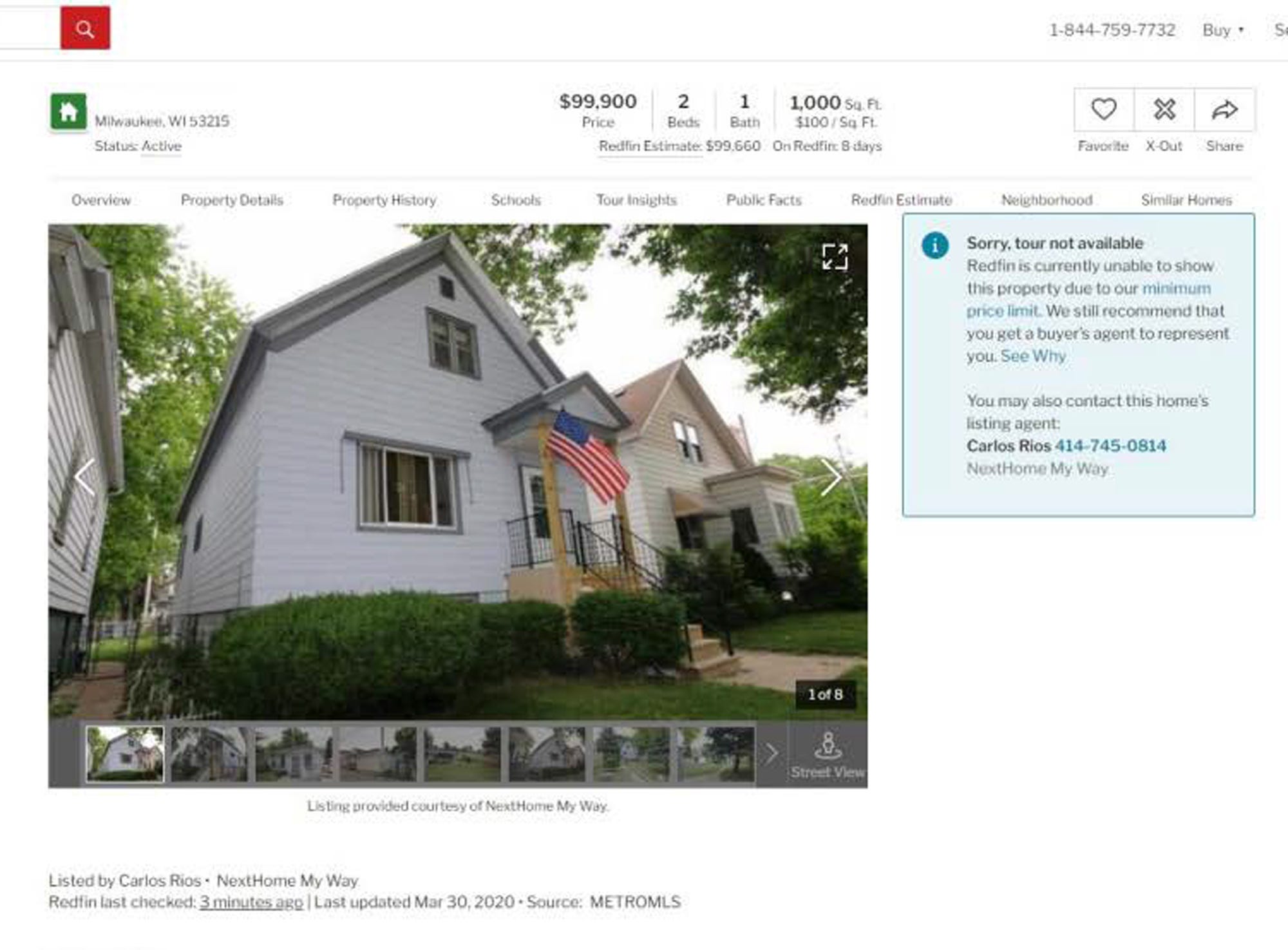This is a listing from a real estate website featuring a property located in Milwaukee, currently active and priced at $99,900. The home includes two bedrooms, one bathroom, and spans 1,000 square feet. 

The main image showcases a modest single-family home painted in white. The house is situated very close to neighboring homes on either side. Leading up to a small entrance that can barely be classified as a porch, there are about nine steps. The entrance features a basic picture window, possibly a small sitting area. 

The house also has a second floor, identifiable by an older-style window with two vertical panes. Below the primary image, there are seven additional images, confirming that this is one of eight photographs available. However, a note on the right side of the main image states that Redfin is currently unable to show a virtual tour due to a minimum price limit.